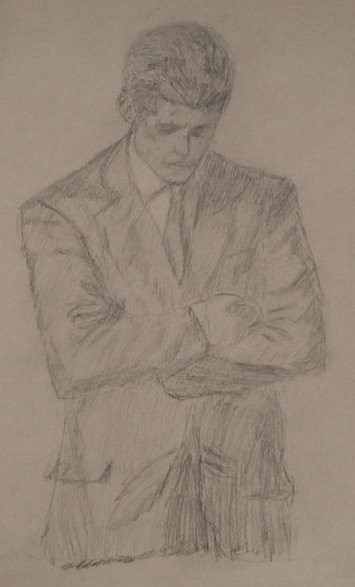This is a detailed pencil sketch on brown craft paper depicting a man from the head to the waist. The man, with his combed-back short hair and clean-shaven face, wears a fitted business suit and tie. His arms are crossed and he is looking down with a somber, almost stern expression reminiscent of JFK. The suit appears well-tailored and emits a sheen, enhanced by the intricate, although somewhat scratchy, pencil shading. Despite the rough texture and varied direction of the pencil strokes, this is a well-executed and striking drawing.